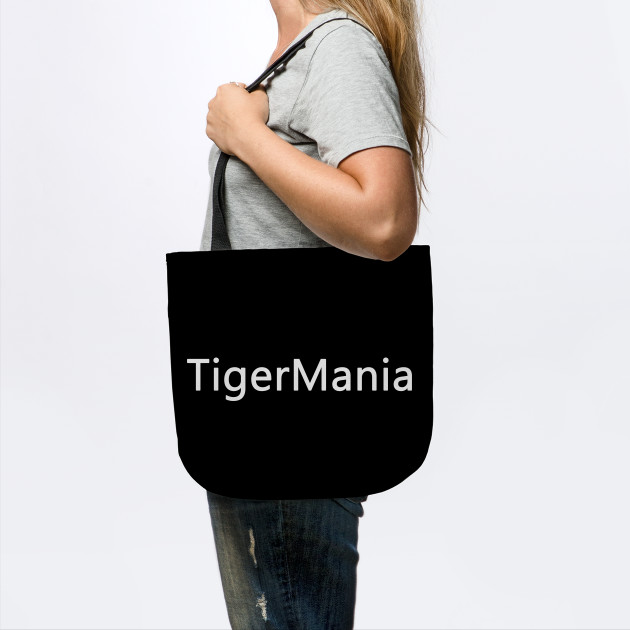A centered image features a Caucasian woman with long blonde hair cascading to her back, wearing a grey short-sleeve t-shirt and slightly distressed blue jeans. Her face and lower legs are not visible, as the image is cropped from just above the knees to the shoulders. She stands facing the left, holding a large black tote bag with a simple black strap draped over her shoulder. The bag, which she holds with her left arm just above her breast, is the focal point of the image. It prominently displays the text "Tigermania" in large grey letters. The plain grey background and the woman's placement in the center emphasize the bag, suggesting it is an advertisement for the bag brand. The overall setting remains ambiguous.